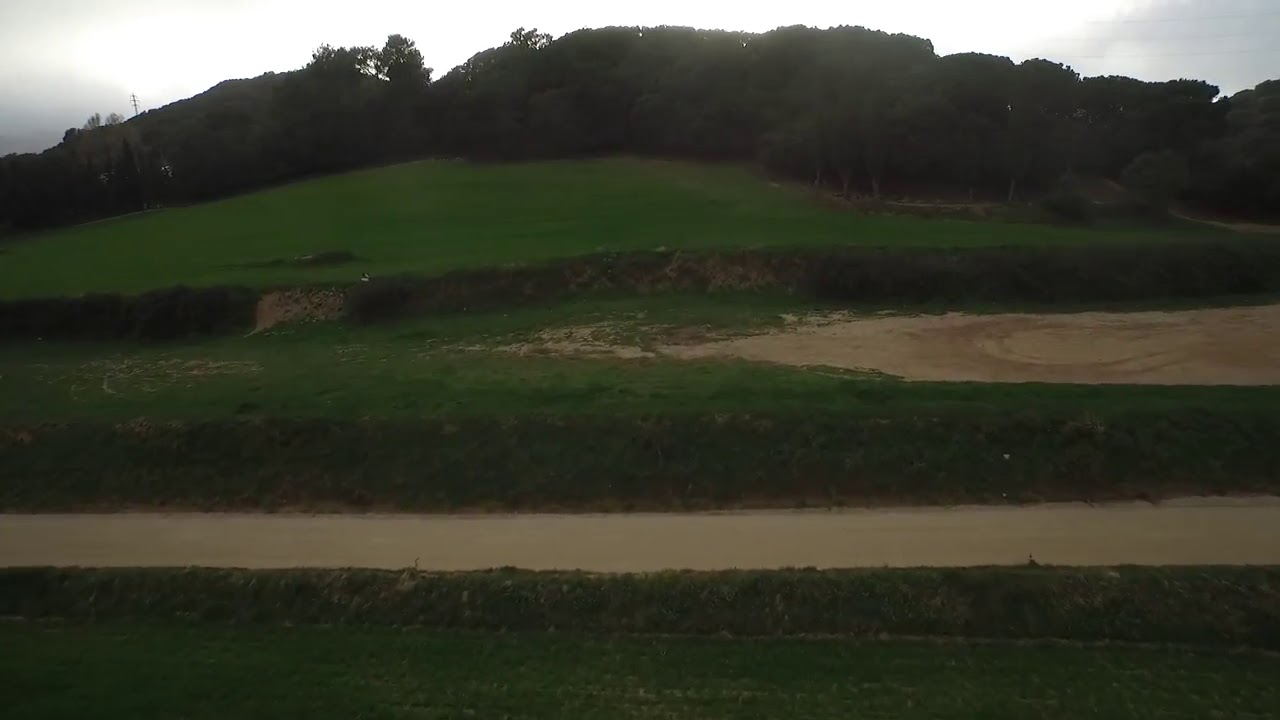The photograph captures a serene outdoor landscape featuring a meticulously terraced grassy hill, suggestive of man-made landscaping rather than natural formation. The hill is divided into distinct levels: the base reveals a beige dirt road or possibly a muddy creek, characterized by its smooth texture and muddied appearance. The second tier consists primarily of tan or sandy terrain, indicating either a dry streambed or a dirt patch. The topmost level is blanketed in lush, green grass interspersed with dark green, mature trees. The backdrop showcases a bright overcast sky with light gray and white clouds, suggesting a partly cloudy day. The overall scene exudes a tranquil yet slightly rugged atmosphere, reminiscent of a reclaimed or repurposed space, such as an old golf course. Dominant colors in the image include green, tan, and white, emphasizing the natural and unembellished beauty of the setting.